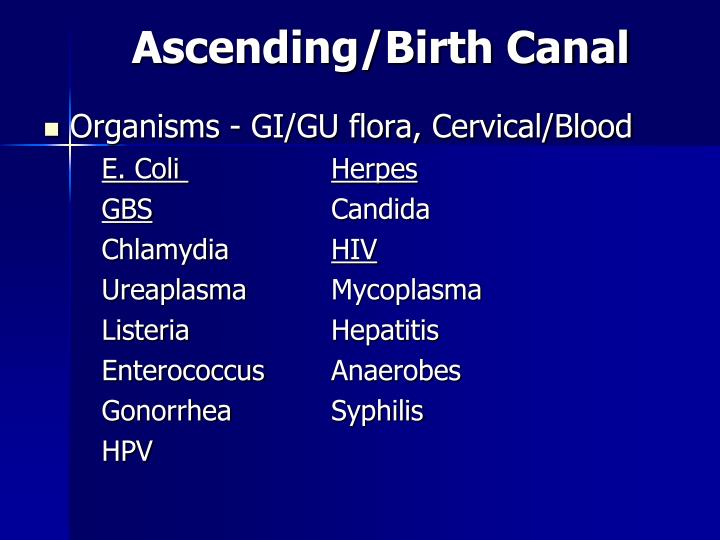The image is a medical PowerPoint slide with a title "Ascending/Birth Canal" prominently displayed at the top center in bold white text against a blue background with various shades. Below the title, in slightly smaller white text, it reads "Organisms - GI/GU Flora, Cervical/Blood." The list of organisms is presented in two columns, detailing several sexually transmitted diseases and other pathogens. The left column lists E. coli (underlined), GBS (underlined), chlamydia, urea plasma, listeria, enterococcus, gonorrhea, and HPV. The right column includes herpes (underlined), candida, HIV (underlined), mycoplasma, hepatitis, anaerobes, and syphilis. The image is formatted simply with white text on a predominantly royal blue background, with an added bit of yellow near the word "organisms."